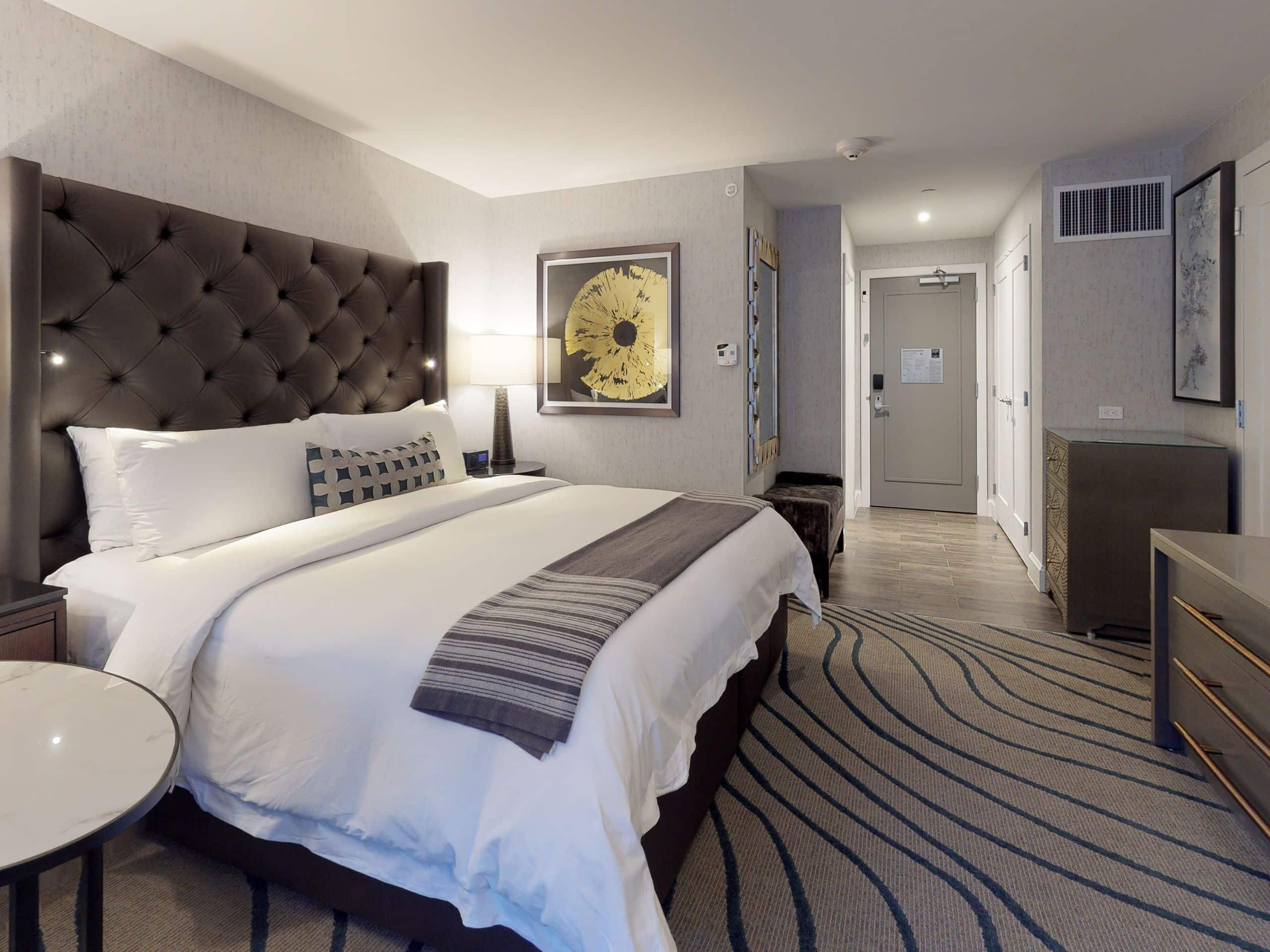The photograph captures a well-appointed hotel room characterized by a harmonious blend of light brown, tan, and black tones. Dominating the center is a king-size bed with an oversized, tufted brown headboard. The bedding includes a pristine off-white coverlet, accompanied by two large white pillows and a distinctive blue and beige crisscross-patterned decorative pillow. Draped at the foot of the bed is a brown and beige striped blanket.

To the left of the bed stands a circular white nightstand, while on the right side, there is a brown nightstand with a black top, both of which feature matching lamps. Above the right nightstand, a painting depicting a flower adds a splash of color to the room, and an air duct lined with white metal is installed above it.

The room features two distinct bureaus: a larger light beige or gray dresser with brass handles and a smaller, intricately embroidered light brown dresser. Near the main entrance – a beige door with a white placard detailing evacuation routes and hotel rates, equipped with a black lock box and silver handle – a small armoire provides additional seating and storage. Above the armoire hangs a mirror partially adorned with miscellaneous items on the left side, adding a personal touch.

The carpet is a neutral tan, intricately designed with blue or black wavy lines. The hallway that leads to the front door is noticeable, emphasizing the room's spacious layout and thoughtful attention to detail. Overall, the design and decor of this hotel room radiate a welcoming, upscale ambiance.